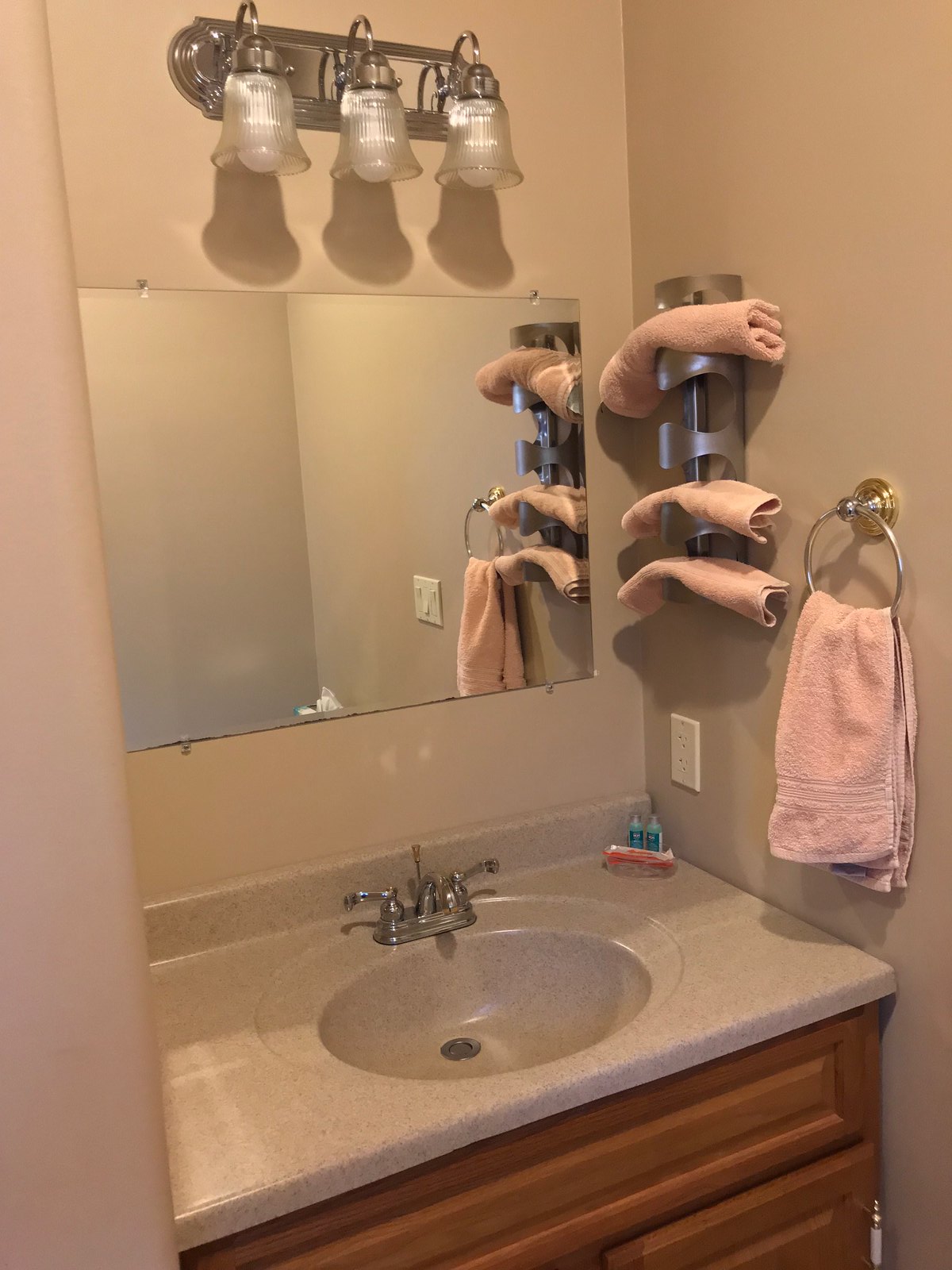This indoor color photograph depicts a pristine, compact bathroom vanity area. The central focus is a small, integrated beige-colored marble sink with a stone basin and a silver, chrome faucet. Below the sink is a vanity cabinet, crafted from light to dark brown wood, featuring two drawers with white handles. On the back wall, a simple mirror is mounted, framed by a beige backdrop. Above the mirror, a light fixture with three downward-pointing bulbs encased in clear glass globes illuminates the area. To the right of the mirror, a silver rack holds three neatly rolled pink towels. Closer to the right edge, a circular hand towel holder hangs a matching pink towel. Additional storage is provided by a wall-mounted shelf, designed to hold extra towels and washcloths. The overall scene is new, clean, and unused, with the walls painted in a coordinating light tan or beige color, and a few shampoo bottles and a soap add minimalistic functionality to the serene setting.